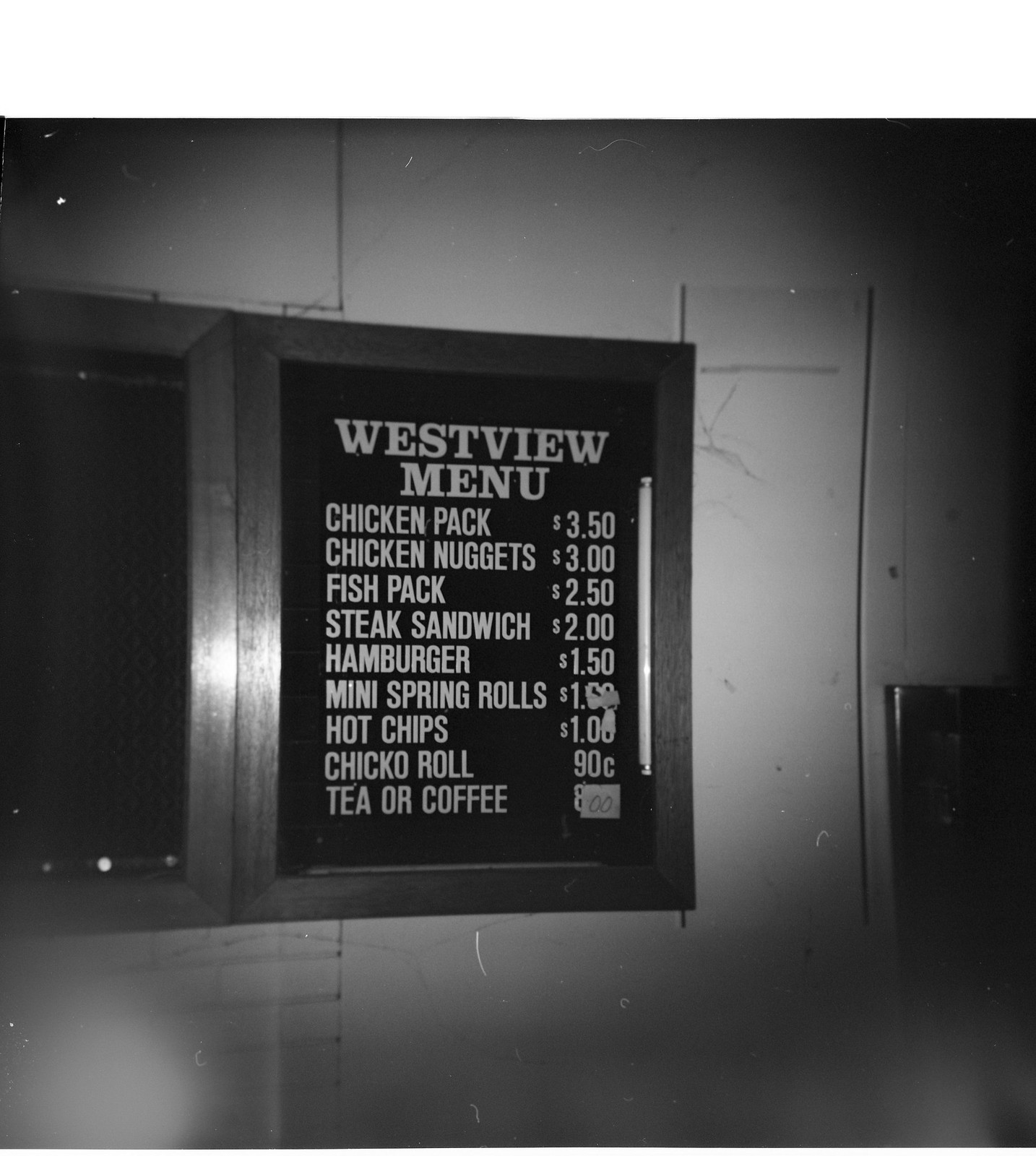In this black and white photograph, a menu is prominently displayed on a white wall. The menu itself appears black with what can be assumed, given the limitations of the black and white photo, to have a brownish border. To the left of this menu is an identical frame, also showcasing the menu but with white text. The title "Westview Menu" is at the top, although it's misspelled as "W-E-S-T-C-I-E-W M-E-N-U". The items listed and their prices are as follows: 

- Chicken Pack (misspelled as "C-H-I-C-K-E-N-D-A-T-C-K") for $3.50
- Chicken Nuggets (repeated as "chicken nuggets, menu E-B-C-C-S") for $3.00
- Fish Pack (incorrectly written as "F-I-C-H C-H-E-K") for $2.50
- Sandwich (spelled as "S-P-E-A-K S-A-M-B-W") for $2.00
- Hamburger (noted as "H-A-M-B-U-R-T-T-R") for $1.50
- Mini Spring Rolls (typed as "M-I-N-I S-P-R-I-N-G R-O-M-P-S") for $1.00
- Hot Chips (listed as "H-O-T C-H-I-C-S") for $1.00
- Chico Roll (written as "C-H-I-C-K-O-R-O-L-L") for $0.90
- Tea or Coffee (noted as "T-E-A-O-R-T-O-S-F-E-E") for $0.00

The various misspellings give the menu a quirky and unique character, adding an element of charm to the scene.